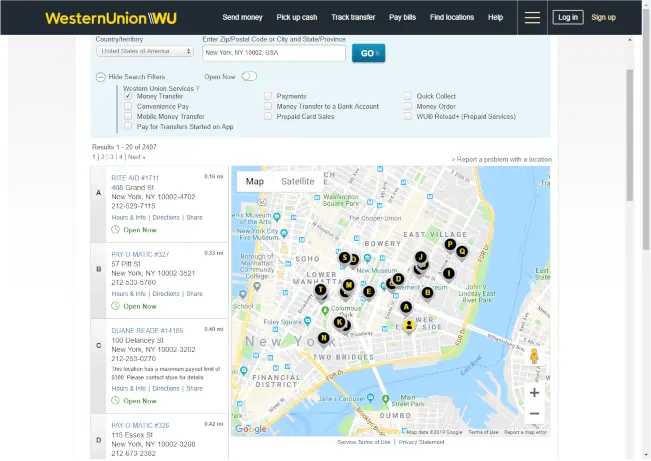The image depicts a web page from Western Union, characterized by its distinctive branding of yellow text on a black background featuring the Western Union logo alongside the letters "WU". To the right of the logo, the navigation menu in white text includes options such as "Send Money," "Pick Up Cash," "Track Transfer," "Pay Bills," "Find Locations," and "Help." Additionally, there are buttons for logging in and signing up.

Below this navigation menu, there is a search interface allowing users to find information by country or territory, with "United States" preselected. Users can also search by entering a zip code, city, or province; the example provided inputs "New York, New York 10002, USA". Adjacent to this input field is a "Go" button to initiate the search.

Further down the page, there are additional search filters that users can toggle to display or hide. The lower portion of the page features a detailed map highlighting various neighborhoods and landmarks in New York City such as East Village, Bowery, New Museum, Lower Manhattan, Two Bridges, and the Financial District. These points of interest are marked with black buttons containing yellow text. Below the map, there is a list of addresses for different locations in New York City.